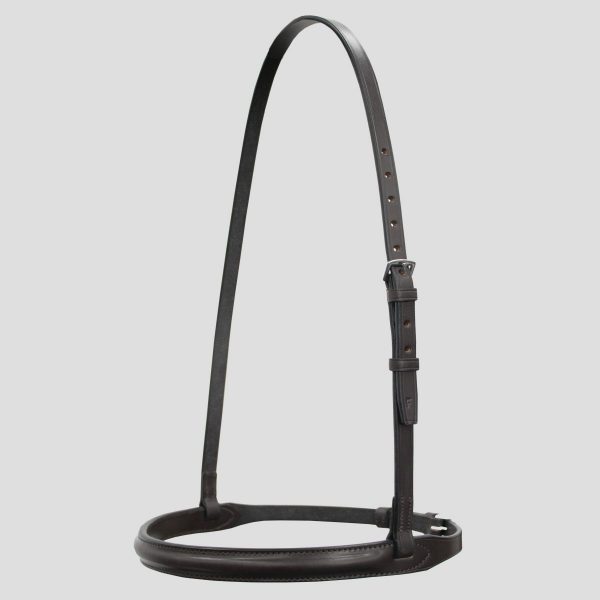A dark brown or black leather belt is prominently featured, suspended in an arch shape. This thin strap, complete with multiple holes and a buckle on its right side, emerges from a circular base. The base, made of either metal or plastic, is a hollowed-out ring with slits on each side serving as attachment points for the belt. The belt loops through these attachment points, creating an upward curve reminiscent of an arch. Despite its supple leather material, the belt maintains this arched form. At the base of the arch, the circular ring provides a stabilizing foundation for the display, which retains a minimalist elegance. The detailed craftsmanship includes visible belt loops and a catch for excess length, hinting at a design that could be part of a sophisticated accessory or functional gear.